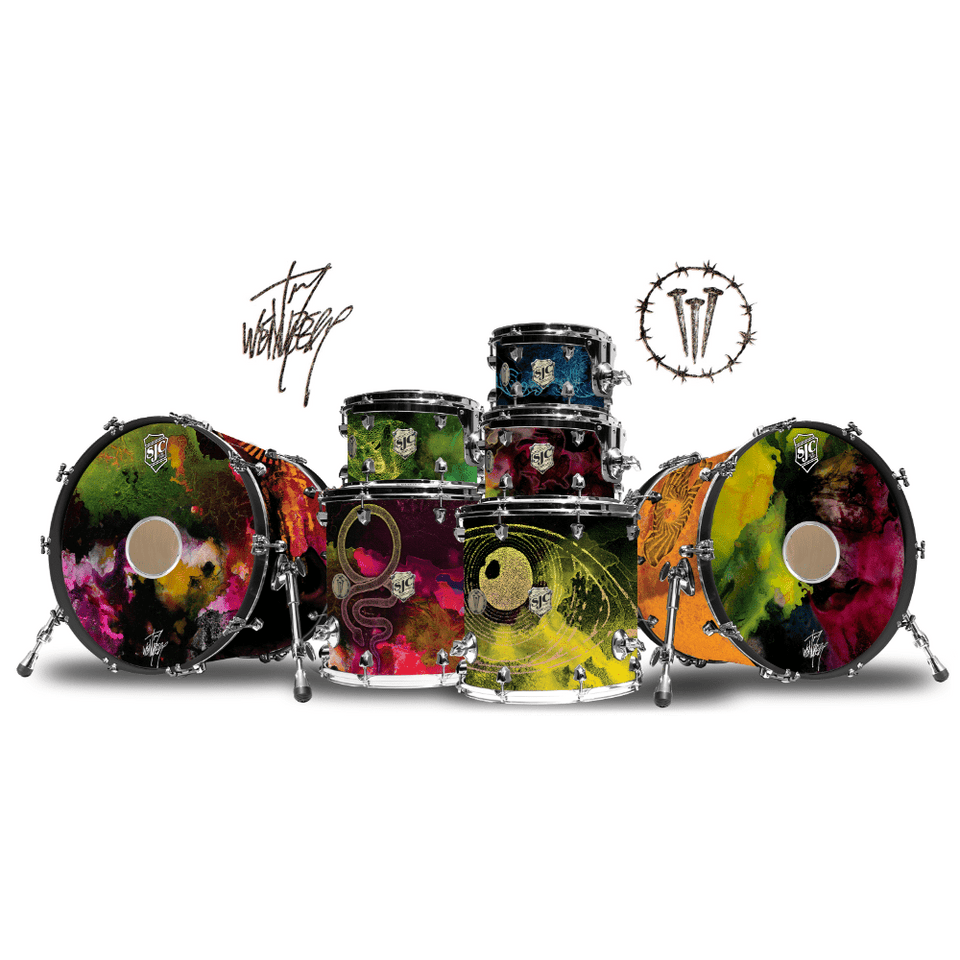The image depicts a vibrantly colorful drum kit on a pristine white background. The drums are arranged in multiple stacks, with two large bass drums flanking the setup. Each drum features an array of jewel-toned colors in a tie-dye style, including reds, purples, greens, oranges, yellows, blues, and pinks, creating a mesmerizing, marbled effect as if the colors are bleeding into one another. The intricate artwork also includes fanciful and trippy designs that adorn the drum skins and sides. On the top left of the image, in black jittery script, is the artist's signature, and to the right, there's a logo resembling a barbed wire circle with three nails inside. The realistic appearance of the drum kit suggests it is a photograph, capturing every detail of the dazzling and chaotic colors on the drum surfaces.